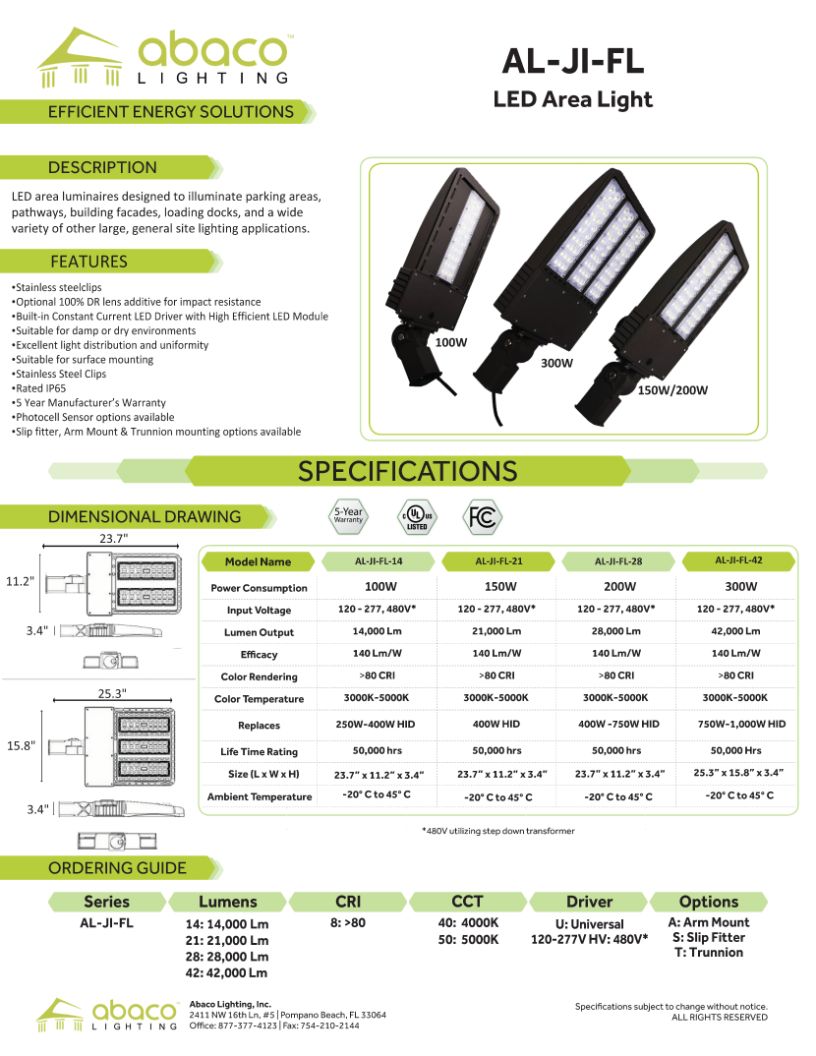This image is a detailed screenshot of the ABACO Lighting webpage. On the left side, the ABACO Lighting logo and company name are prominently displayed. At the top right, the header reads "LGPHIL, LED Area Light." Below, a description succinctly explains that these LED area luminaires are designed to illuminate parking areas, pathways, building facades, loading docks, and various other large general site lighting applications.

The feature section highlights numerous attributes of the LED lights. Adjacent to this text is a photograph showcasing three different lights with varying wattages: 100 watts, 300 watts, and a dual option of 150/200 watts. Beneath the photo, there is a specifications section, detailed with intricate information on the product's dimensional drawings and associated sketches to the left.

To the right of the sketches, the specifications cover aspects such as model name, power consumption, input wattage, lumen output, efficacy, color rendering, color temperature, replacement equivalency, lifetime rating, size (dimensions in length by width by height), and ambient temperature, organized into four columns for different product comparisons.

At the bottom of the page, there is a tab for the ordering guide which includes the physical address of ABACO Lighting along with the office phone number, fax number, and a note indicating that all rights are reserved.